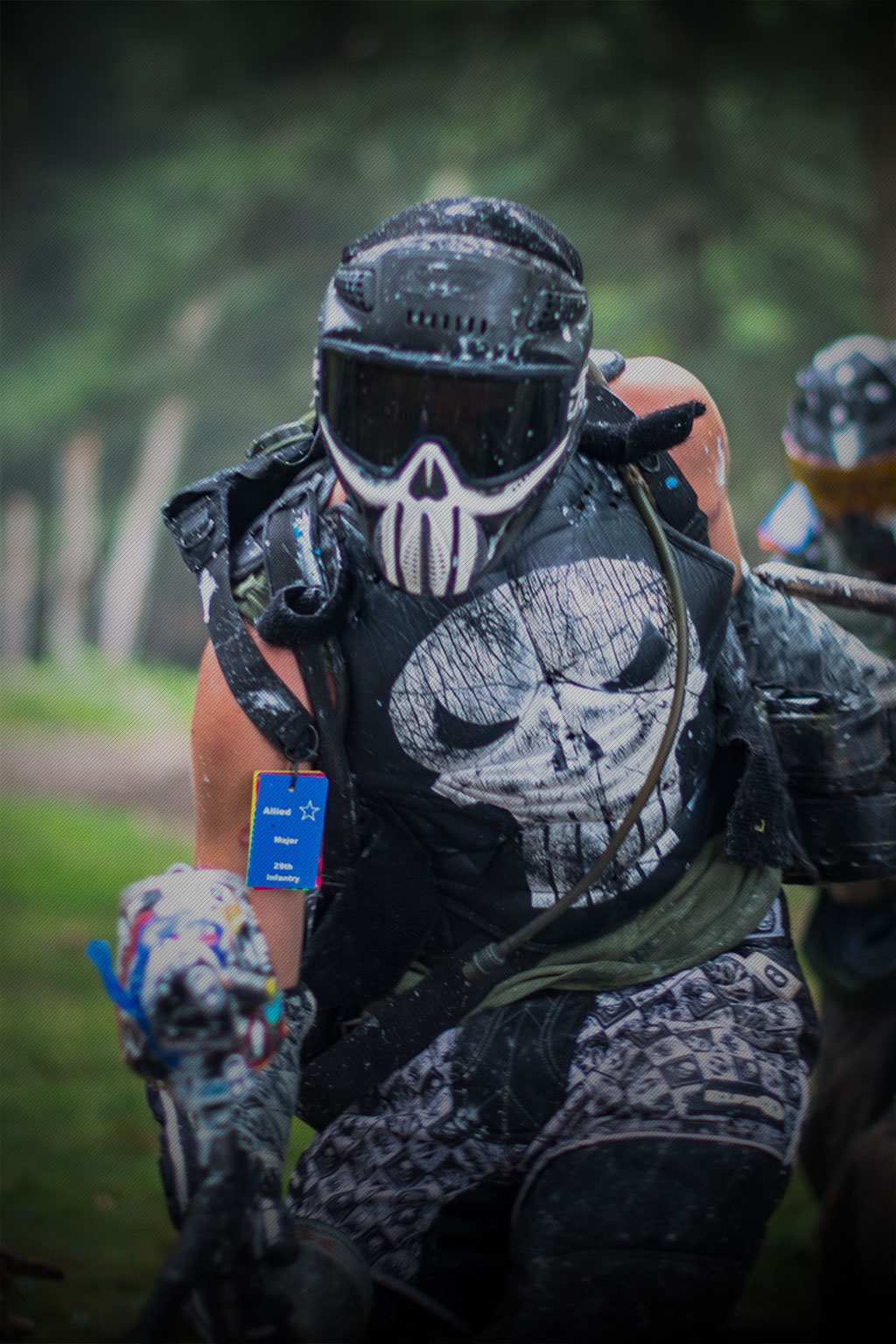This color photograph, in a portrait orientation, captures a dynamic scene of a paintball player actively engaged in a paintball battle. The primary subject is a person facing the viewer, clothed in gothic attire. They are wearing a weathered black helmet with a chipped top and attached black goggles that obscure their face, featuring a distinct white skull design along the bottom resembling a goatee. Their sleeveless black shirt, adorned with a white skull on the front, has several horizontal lines descending from the skull, complemented by a protective black vest made from thick rubber. This vest also bears a similar skull motif.

Additionally, the player is equipped with a paintball gun in their right hand, intricately detailed with various paint splatters in multiple colors, and a tube leading from the gun to a backpack likely containing their air supply. A blue tag is visible on one of the straps. The player is dressed in black pants with denim shorts worn over them, possibly for extra protection. Over their right shoulder, the head of another player can be seen, partially visible.

The background comprises a forested scene or mural in shades of green and brown, slightly out of focus, emphasizing the energetic realism of the scene.